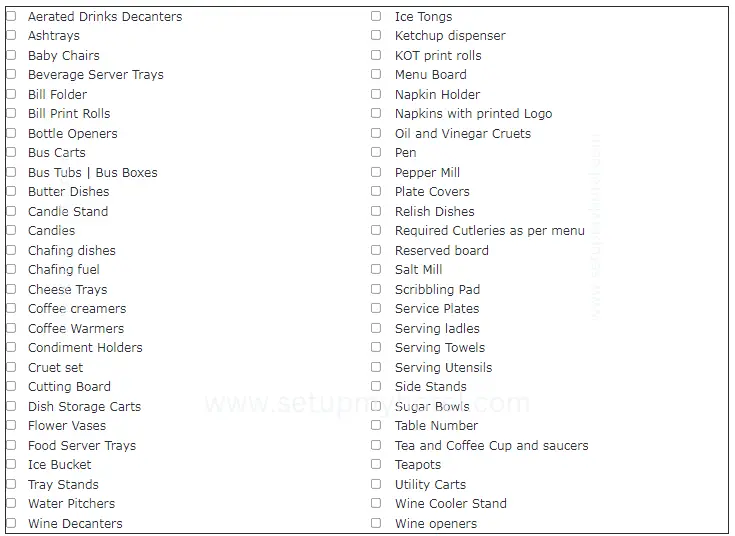In this image, we see a detailed inventory list divided into two vertical columns, each containing various categories of hospitality items. 

On the left column, from top to bottom, are: 
- Aerated drinks decanters
- Ashtrays
- Baby chairs
- Beverage server trays
- Bill folders
- Bill print rolls
- Bill bottle openers
- Bus carts
- Bus tubs
- Water dishes
- Candle stands
- Candles
- Chafing dishes
- Chafing fuel
- Coffee creamers
- Cheese trays
- Coffee warmers
- Condiment holders
- Crust sets
- Cutting boards
- Dish storage carts
- Flower vases
- Food server trays
- Ice buckets
- Tray stands
- Water pitchers
- Wine decanters

Each of these categories includes a small square with a gray outline to the left, which can be checked off.

The right column, from top to bottom, includes:
- Ice tongs
- Ketchup dispensers
- KOT print rolls
- Menu boards
- Napkin holders
- Napkins with printed logo
- Oil and vinegar cruets
- Pens
- Pepper mills
- Plate covers
- Relish dishes
- Required cultures as per menu
- Reserved boards
- Salt mills
- Scribbling pads
- Service plates
- Serving ladies
- Serving towels
- Serving utensils
- Side stands
- Sugar bowls
- Table numbers
- Tea and coffee cups and saucers
- Teapots
- Utility carts
- Wine cooler stands
- Wine openers

All category names are written in black text against a white background, which provides a clear and organized layout for easy reading and management.